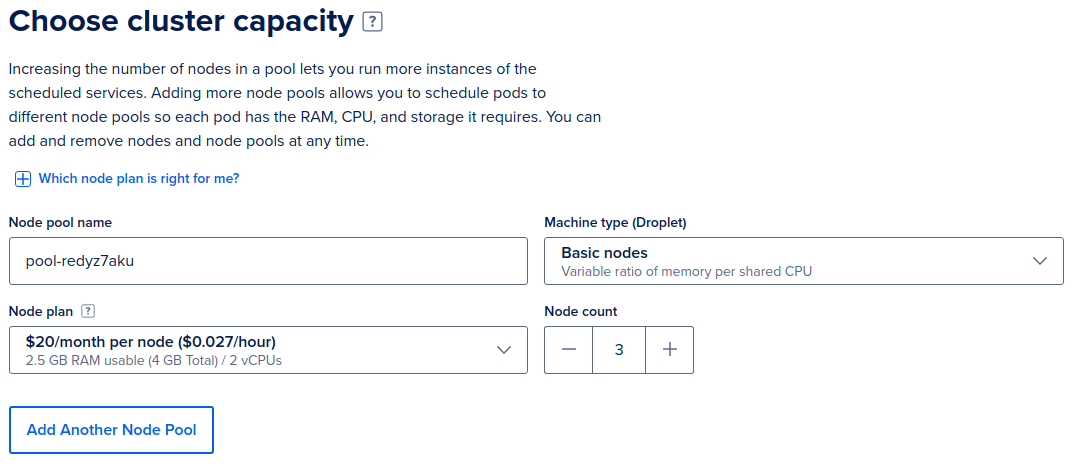Screenshot Description: Cluster Capacity Configuration Interface

The screenshot depicts a user interface for configuring cluster capacity, featuring a clean, minimalist design with a pure white background. The heading, "Choose Cluster Capacity," is displayed prominently at the top in big, bold Myriad font. Below this heading, a detailed explanation informs the user about the importance of increasing the number of nodes: "Increase the number of nodes in a pool to run more instances of the scheduled services. Adding more node pools allows you to schedule pods to different node pools, ensuring each pod has the RAM, CPU, and storage it requires. You can add or remove nodes and node pools at any time."

One of the prominent interactive elements is the blue text with a plus symbol labeled "Which node is right for me." This indicates a clickable link or expandable section offering assistance in selecting the appropriate node.

The interface contains several input fields, each with specific labels:
- **Node Pool Name:** This field likely allows users to name their node pool for identification.
- **Machine Type:** Dropdown or selectable options for choosing the machine type.
- **Droplet:** An option within the machine type selection.
- **Node Plan:** Detailed pricing information is provided, stating "$20 a month per node or $0.027 an hour."

The interface displays the current node count as "3," indicating the user has selected three nodes for the cluster.

At the bottom of the screen, there is a blue box labeled "Add Another Node Pool," allowing users to easily expand their cluster capacity by adding more node pools.

The entire screenshot is captured within an unidentified application, as no specific branding or app name is visible. The design focus remains on functionality and user guidance, with clear instructions and straightforward options for managing cluster resources.